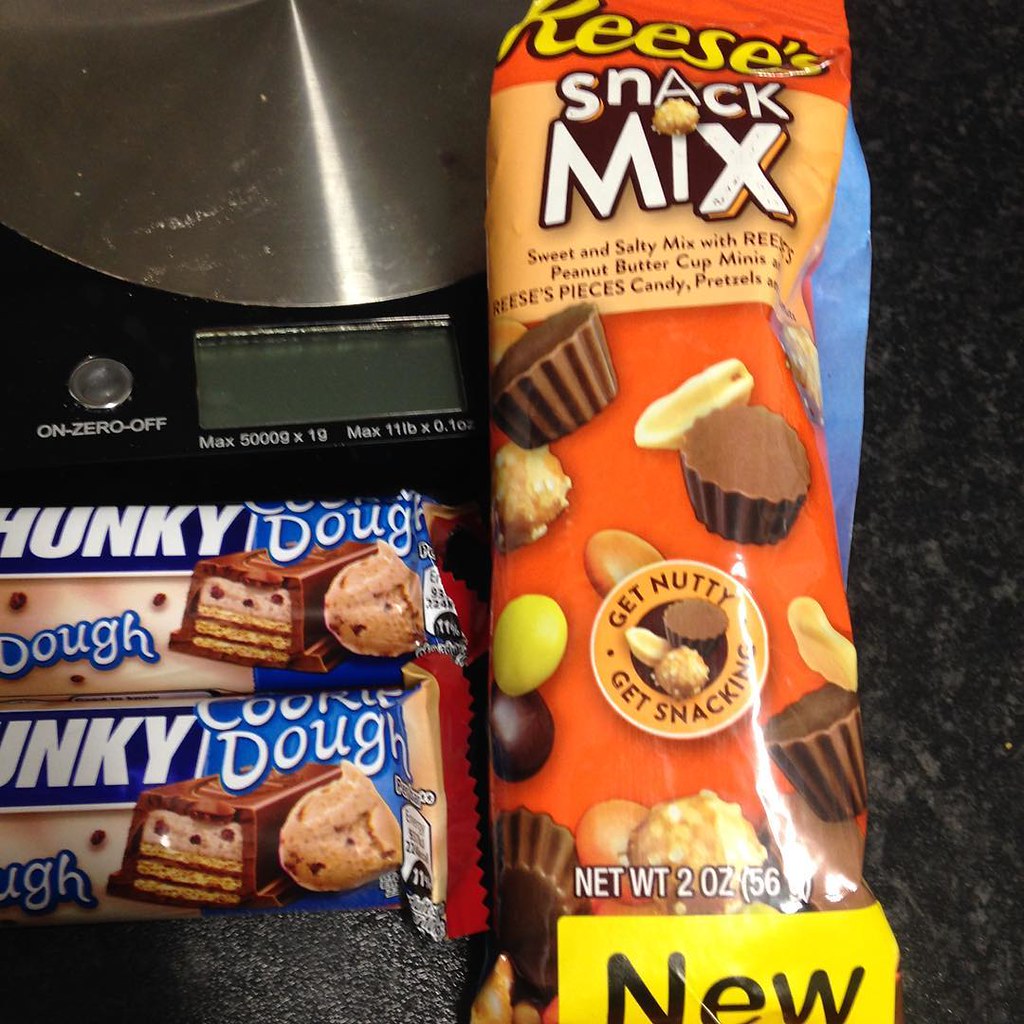The image features a digital scale in the upper left corner, which is black with a round center piece and an inactive digital display. Below the scale, on a black counter, are two horizontally-placed candy bars with white, blue, beige, and red packaging, bearing the words "chunky" and "cookie dough," and featuring an image of rectangular-shaped chocolate bars. To the right of these candy bars is a vertically-standing orange package labeled "Reese's Snack Mix." The wrapper details a sweet and salty mix containing Reese's Peanut Butter Cup Minis, Reese's Pieces, and pretzels, with pictures of the candy throughout. The wrapper also states the net weight as 2 ounces (56 grams) and highlights the product as "new."